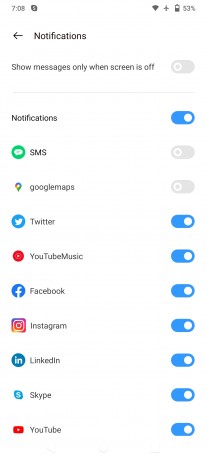The image depicts a screen designed for configuring specific notifications on a device. At the very top, the option "Show messages only when the screen is off" is displayed but currently disabled. Below this, a fine grey line separates the top section from a list of specific notification settings.

These settings include:
- **Notifications:** Enabled, indicated by a blue slider positioned to the right.
- **SMS:** Disabled.
- **Google Maps:** Disabled.
- **Twitter:** Enabled.
- **YouTube Music:** Enabled.
- **Facebook:** Enabled.
- **Instagram:** Enabled.
- **LinkedIn:** Enabled.
- **Skype:** Enabled.
- **YouTube:** Enabled.

At the top of the screen, the current time is shown as 7:08. To the right of the time, there are several small icons, including one resembling an upside-down diamond, likely indicating WiFi status, a plane symbol for flight mode, and a battery icon showing a 53% charge.